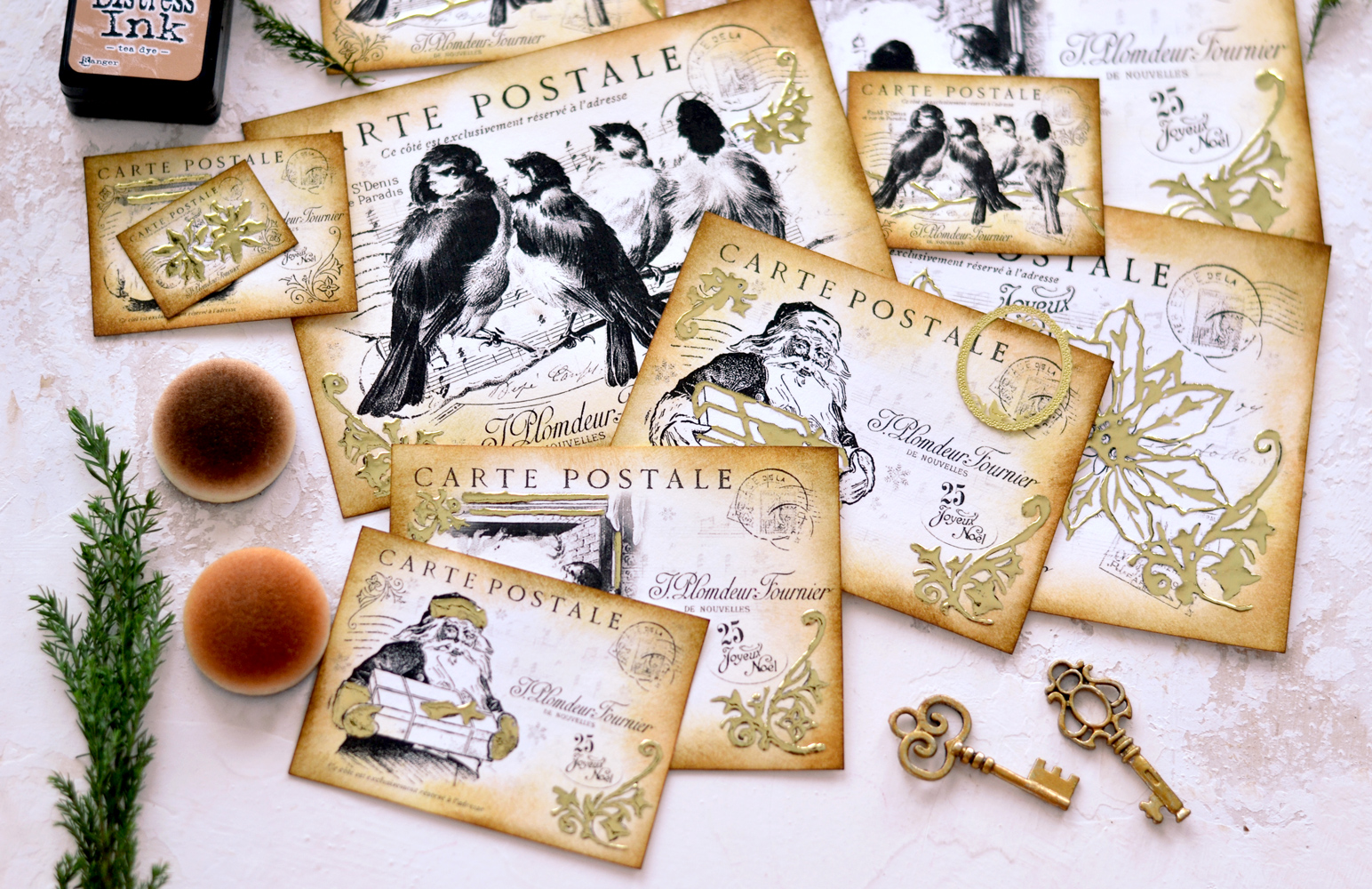The image depicts a collection of vintage-style postcards scattered across a white surface. Dominating the center are around a dozen postcards of varying sizes, predominantly featuring black-and-white illustrations with brown, aged edges. Many of these postcards display the title "Carte Postale" in a foreign script. The prominent designs include Santa Claus holding a rectangular gift and several postcards topped with black and white birds. 

On the upper right, there's a package labeled "Basic Inks," suggesting accessories perhaps from a postcard or stamp crafting kit. In the bottom right corner, two antique bronze keys rest, adding to the old-timey aesthetic. To the left side of the image, a vibrant sprig of green foliage contrasts with the otherwise muted colors and two small brown buttons or spheres can be seen nearby. An air of vintage charm and creative craftiness pervades the scene, hinting at a personalized or handmade postcard project.